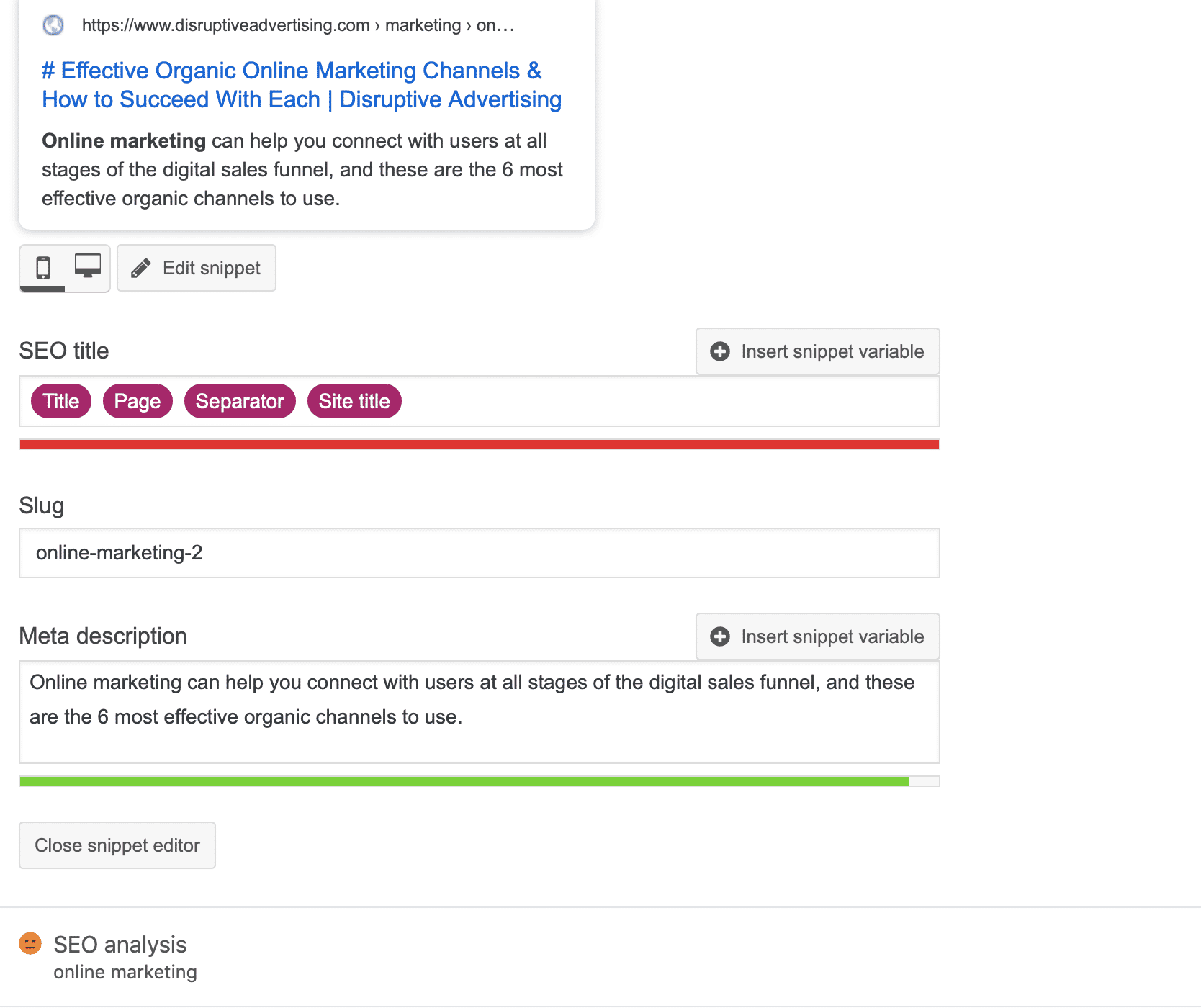Screenshot of the Disruptive Advertising website with a white background. In the upper left corner, there's a white rectangle containing a small gray globe icon, followed by the URL "https://www.disruptiveadvertising.com" in black font. Below this, a blue font reads "Effective Organic Online Marketing Channels and How to Succeed with Each" adjacent to a vertical blue line. The text "Disruptive Advertising" appears after the line.

Further down, in black font, it states: "Online marketing can help you connect with users at all stages of the digital sales funnel, and these are the six most effective organic channels to use."

Below this section, there are two small gray rectangles. The left rectangle features an icon of a smartphone and a computer monitor, and the right rectangle displays an icon of a pencil in black font. To the right of these icons, the text reads "Edit Snippet." Finally, below this, another line of black text says "SEO Title."